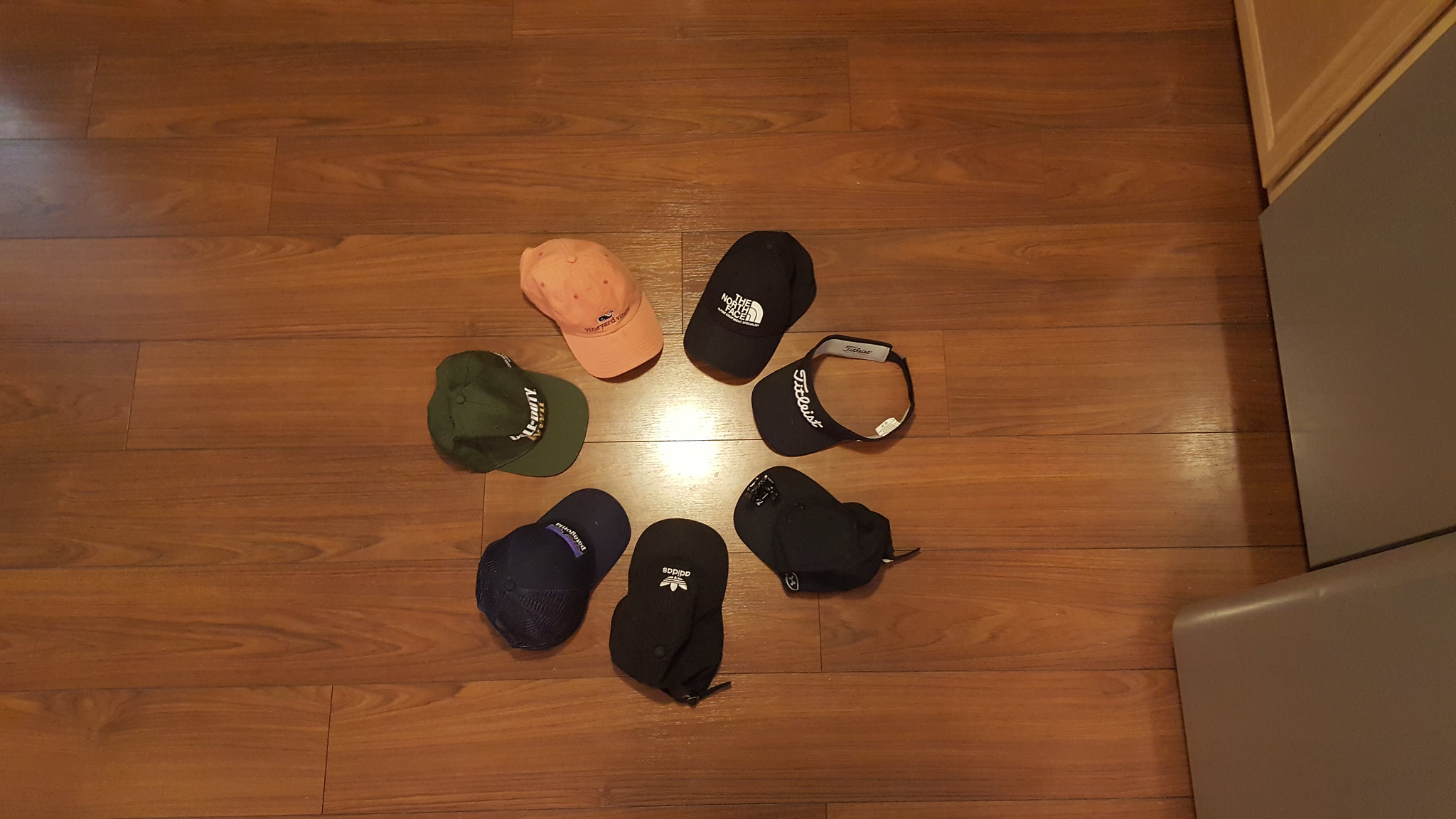This top-down photograph captures an arrangement of seven hats, including one visor, meticulously positioned in a circular pattern with their bills facing inward, mimicking the rays of the sun. They are set on a dark brown, wooden panel floor inside a home, showcasing the wood's natural grain. The hats are evenly spaced, creating a visual effect reminiscent of a sun with shining rays originating from a central point, which appears to be the reflection of a light source above or the camera itself. 

The collection of headwear features a variety of colors: four black hats, one green, one navy blue, and one beige or peach-colored hat. Most of the caps have white writing or symbols on them, with specific details visible on some; for example, one black cap bears the logo for The North Face, and another black cap features the Adidas logo. The visor is also black with white writing. 

In the right-hand portion of the image, elements of the indoor setting are visible, including a grayish wall with a smooth texture and part of a light brown door located in the top right corner. The photograph, rectangular in shape, cohesively captures this artistic hat arrangement in a home interior setting.